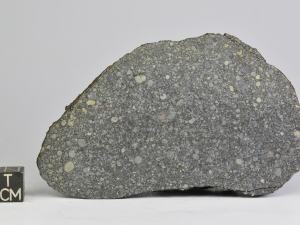This landscape photograph features a large, oval-shaped quartz rock sliced in half, revealing its intricate interior. The rock's exposed flat side showcases various shades of charcoal gray interspersed with lighter gray and white sub-circles, all set against a subtle, off-white background. The rock's outer surface retains a crusty, textured appearance, tapering to a thin, lumpy ridge along its left and right edges. The left, top, and bottom sides of the rock are fully visible, while the right edge is cropped by the picture's frame. In the lower left corner, a small black cube displays the white-etched text "TCM." Shadows cast by the rock emphasize its dimensionality against the minimalist background. No other elements, colors, or text intrude upon this focused composition.